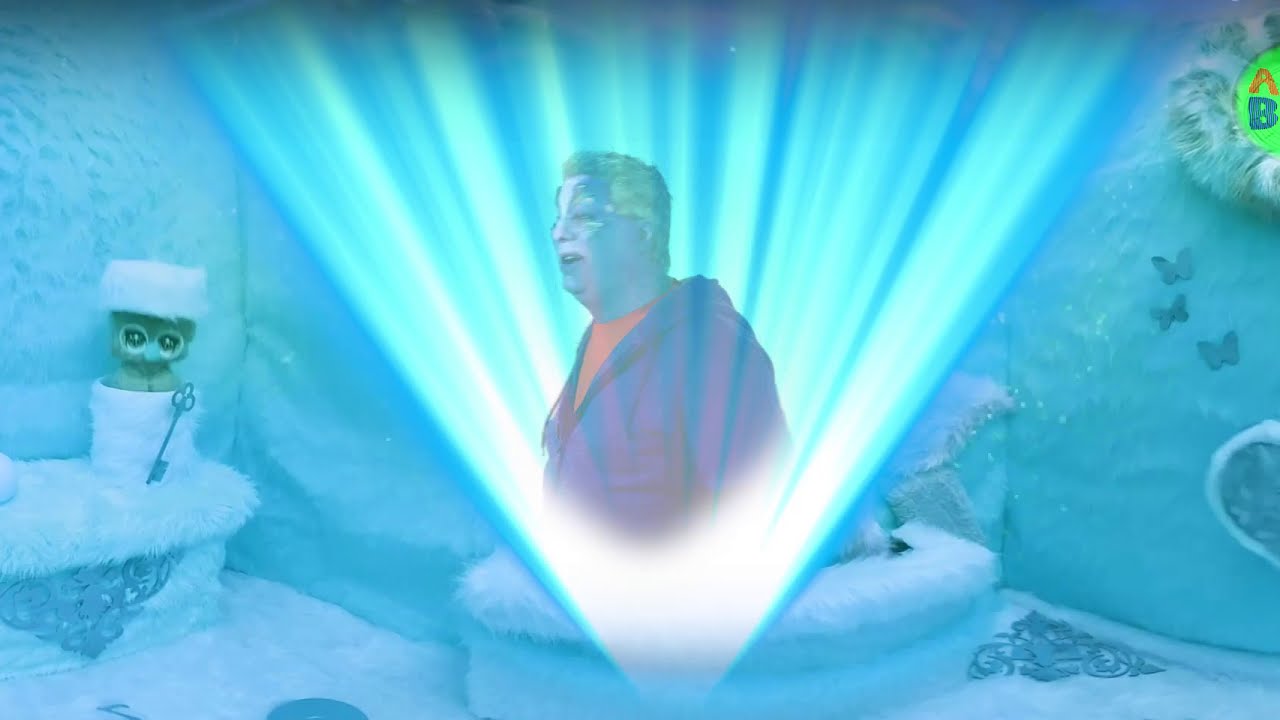In this unusual and graphic collage-like image, the central figure is a middle-aged man, visible from the waist up, who commands attention. He has blonde hair and his face is painted with black makeup from the nose upwards, giving him a striking appearance with squinted eyes and an open mouth showing a double chin. He wears an orange shirt under a blue hoodie. The man, semi-transparent and evocative of Rodney Dangerfield, gazes off to the left while standing amidst a surreal environment. Radiating from the bottom-center of the image is an upside-down, triangular beam of light, bright at its base and fanning outwards to the top corners, framing the man both in front and behind.

The backdrop is a whimsical, fairy-tale-like room with textured, fluffy, white and bluish walls adorned with butterflies. Amidst this scene is a small, white, furry cup with a baby owl peeking out and a key placed in front of it. Additionally, there is a strange creature inside a small box on the left side. On the right, a neon green semi-circle bears the letters "A" and "B" in red and blue respectively. The floor appears snowy and furry, adding to the dreamlike quality of the image. The overall color scheme is dominated by whites, blues, and greens, creating an ethereal yet perplexing setting.